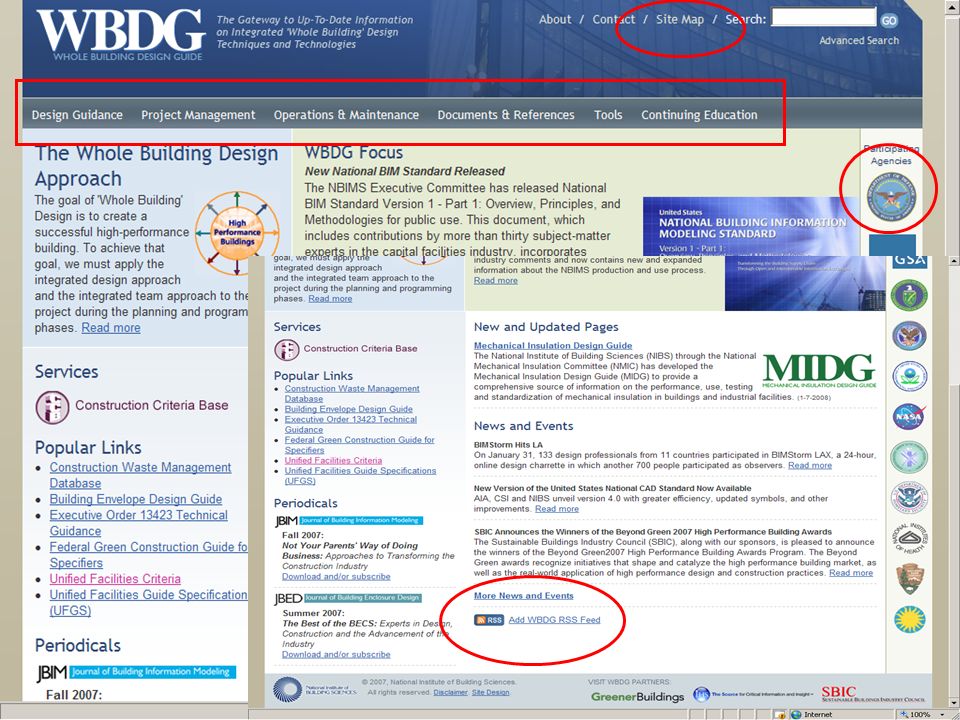This image, sourced from the Whole Building Design Guide (WBDG) website, showcases a well-structured layout aimed at providing comprehensive building design resources. At the top of the screen, a blue banner is prominently displayed, followed by a navigation bar with several tabs including "About," "Contact," "Site Map," and "Search." Notably, the "Site Map" tab is encircled with a red outline, emphasizing its importance, while a white search box is positioned for users to type in queries for additional information.

Below the main navigation, a secondary set of tabs is outlined in a red square, offering a range of categories such as "Design Guidance," "Project Management," "Operations and Maintenance," "Documents and References," "Tools," and "Continuing Education," thereby facilitating easy access to specific information.

Moving down to the body of the webpage, the focal area is filled with textual content. On the left side, a section titled "The Whole Building Design Approach" catches the viewer's attention. The introductory text explains that the goal of whole building design is to create a successful high-performance building. It emphasizes the necessity of applying both the integrated design approach and the integrated team approach during the project's planning and programming phases. A "Read More" link, highlighted in blue and underlined, invites users to click for further details on the whole building design approach, allowing for deeper exploration of the subject.